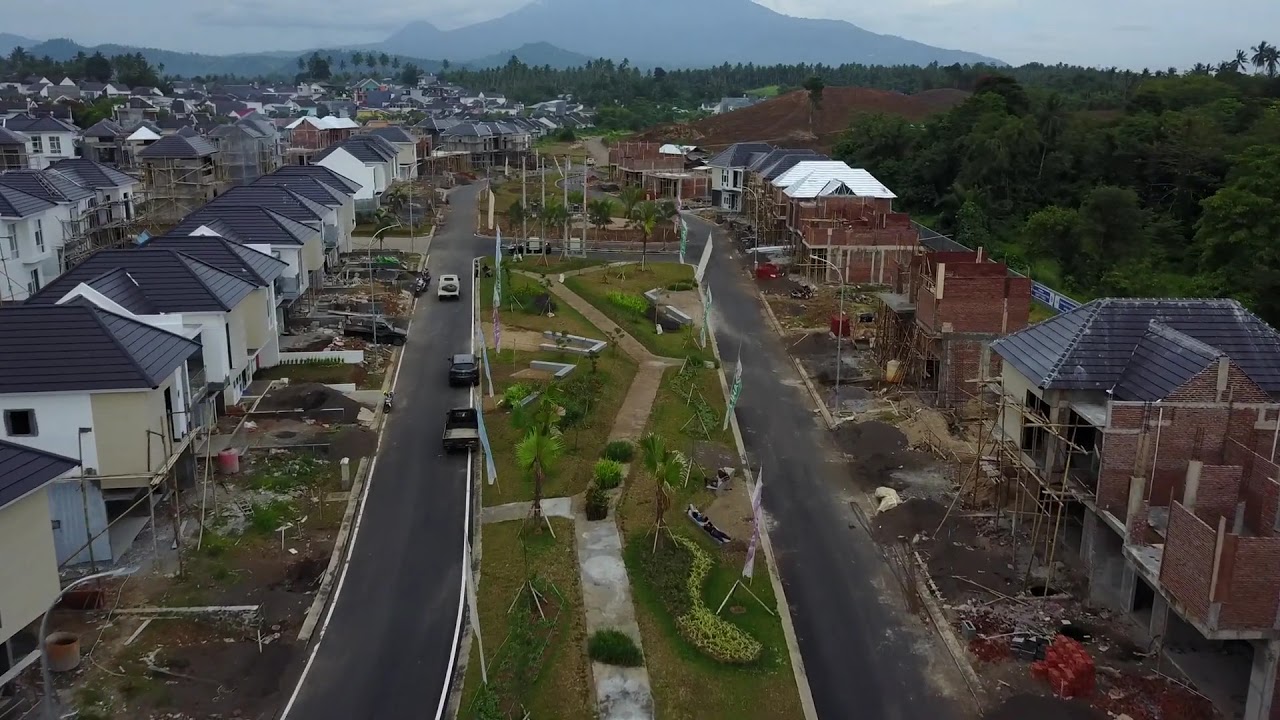This aerial photograph, likely taken from a drone during the daytime, captures an expansive construction site nestled between a forested area and towering mountains under a grayish-blue sky. The image prominently features two parallel rows of houses in various stages of construction. On the left side, a row of white houses with black roofs stands amid a chaotic array of construction vehicles and equipment, with minimal landscaping and clear signs of ongoing work. In front of these houses, a street runs parallel to a central green median that functions as a park area. This median includes a walkway with shrubbery still in pots and newly planted trees stabilized by wooden tripods. On the right side of the image, another row of homes is being constructed, these predominantly red-brick structures are less complete, with many still bare frameworks and scaffolding in place. The scene is framed by lush greenery and a line of trees, set against the backdrop of imposing mountains, highlighting both the natural beauty of the surroundings and the industrious activity of the development.